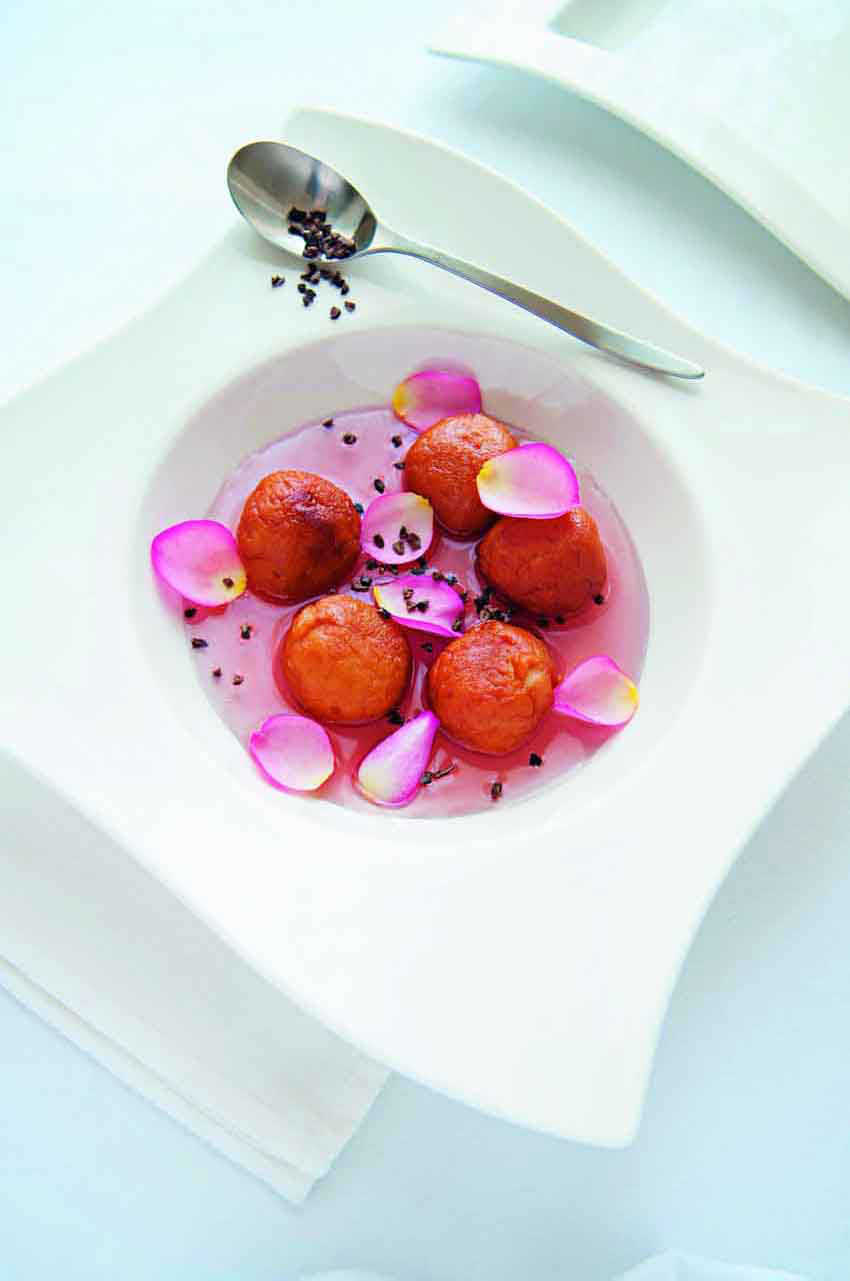The photograph, taken indoors, features a distinctive white bowl with wavy, square-ish edges and a flat, plate-like rim. Centered within the bowl is a pink liquid, hinting at a reflection of pink petals floating atop and mixed within the fluid. Suspended in the liquid are several sphere-shaped fruits, possibly passion fruits, mistakenly presumed to be strawberries but without seeds. Sprinkled around and on these fruits, as well as within a metal spoon resting on the bowl's ledge, are black speckles, potentially pepper or black sprinkles. Additionally, rose petals in shades of pink or purple add a delicate touch to the composition. The bowl and spoon ensemble rests on a light blue table with a white napkin visible in the lower left corner. In the background, another similar bowl or plate is partially seen in the top right corner, its contents indiscernible. The entire scene portrays an artfully arranged culinary presentation.